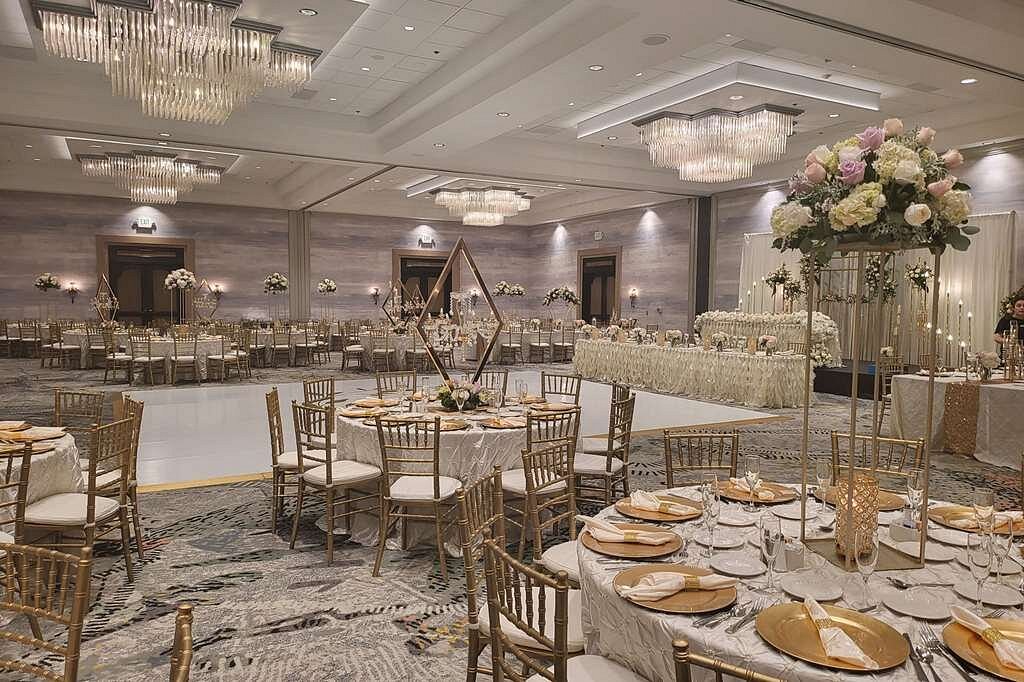This image captures a grand wedding reception held in a spacious, ornate ballroom. The high, white ceiling, adorned with intricate molding and four or more chandeliers that hang like blocks of icicles, occupies the top third of the frame. The chandeliers cast a soft glow over the elegantly set scene below. The spacious room features wood-paneled walls with horizontal slats in a light wood color, and large, French-style, brown doors that open out into the room.

The dining area is composed of multiple round tables dressed in pristine white tablecloths, set on black and white printed rugs. Each table is adorned with bronzed or golden plates, complete with white napkins held by gold bands. Tall wine glasses and smaller salad plates complement the settings, while the centerpiece on each table boasts a tall, bronze stand topped with a bouquet of vibrant hydrangeas, roses, and other flowers in shades of light pink, peach, and white. Beneath these floral arrangements, candles flicker, adding to the romantic ambiance.

In the center of the room, a long table on a raised stage is also decorated with white flowers and candles of varying heights, crowned by a tall central candle. This table, likely for the bride and groom, is backed by an elegant white draping. In front of this main table lies a large, white dance floor, hinting at the celebration's festivities. 

A centerpiece table features an inverted square stand, elegantly displayed on one of its points, with a flower arrangement beneath it. Nearby, a person, possibly a server, is partially visible on the right side of the image. Overall, the meticulous and ornate decorations, along with the detailed setup, suggest a lavish wedding reception in full swing.